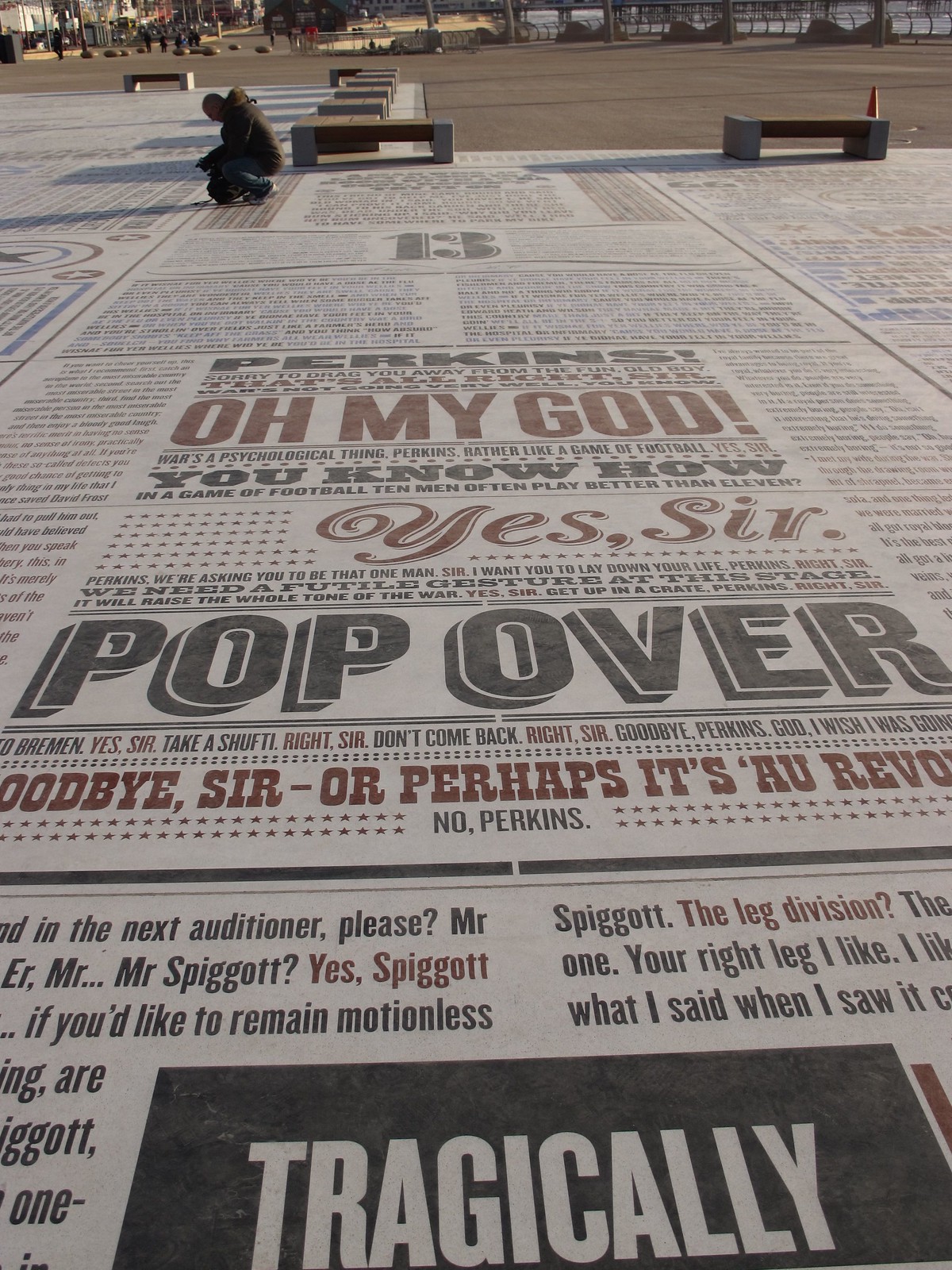This photograph taken outdoors captures an expansive concrete area adorned with benches along the sides, where the ground serves as a canvas for a sprawling, newspaper-like print. The printed text, in stark black and white with occasional touches of red, features fragmented phrases such as "Perkins," "Oh my God, you know how?" and "Yes sir, pop over, goodbye sir." Toward the bottom of the image, a black rectangular box contains the word "TRAGICALLY" in bold, white uppercase letters. Other visible snippets of text include peculiar phrases like "spigot" and "the leg division." The area appears almost surreal, as it's uncommon to see ground covered in such extensive writing. Kneeling near the top left of the frame is a person in a brown coat, absorbed in reading the text. Distant elements like dirt, trees, housing, and a parking lot can be spotted, along with a traffic cone. The overall scene evokes a sense of mystery, perhaps hinting at a memorial or an art installation.